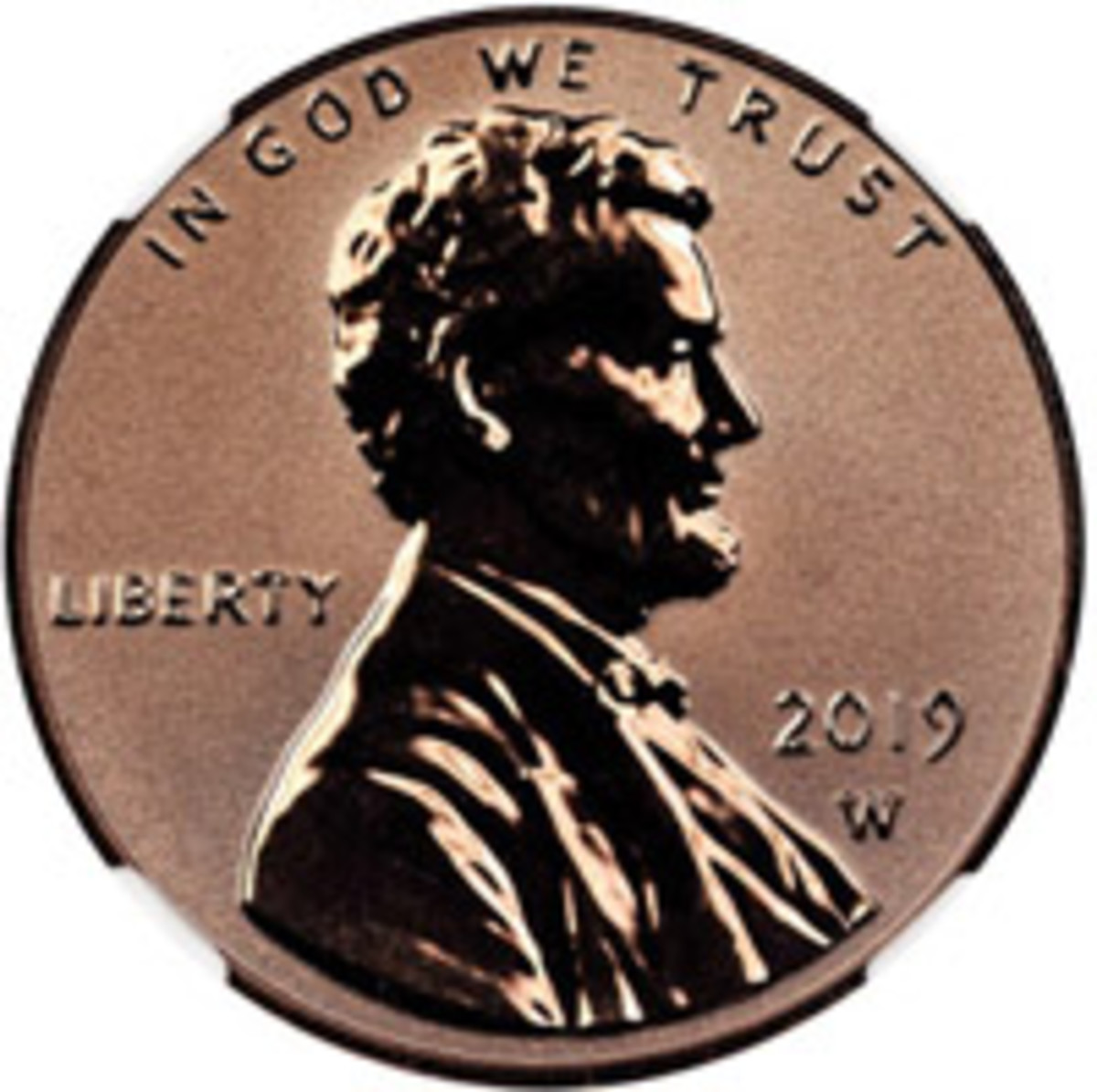This highly magnified and somewhat out-of-focus image features an American penny, with clear indications that it has been expanded beyond its natural resolution. The background is a featureless white, highlighting the penny, which stands out in its copper or bronze hue. The design includes the standard profile of Abraham Lincoln, who is depicted facing sideways with distinct hair and a suit. The words "In God We Trust" are prominently displayed above Lincoln's head, while the word "Liberty" is positioned to his left. The mint mark "2019 W" is located at the bottom right, indicating it was minted in West Point. The lighting appears oblique, casting bright highlights and deep shadows across Lincoln's face, suggesting the light source is from the left. Notably, the penny shows damage or manipulation around its edges, with four areas along the rim suggesting it was once held by prongs in a display, which have since been photoshopped out.